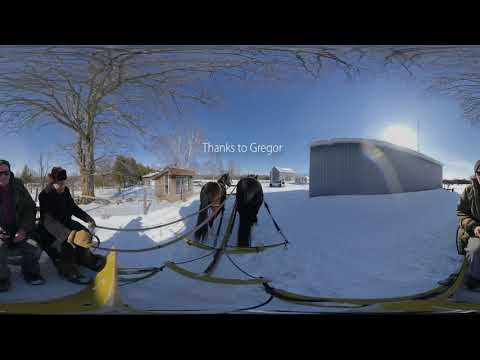In this snowy outdoor scene, a group of people appears to be enjoying a ride on a yellow sleigh pulled by two horses, one black and the other brown. These horses, positioned in the center of the image, have the words "thanks to Gregor" written above them. Despite the slightly blurry quality of the image, the blue sky and the sun shining in the top right corner are clearly visible. 

On the left side of the image, two men are seated on the sleigh. The man on the right is holding onto both sides of the sleigh, which is secured with black ropes. He is dressed in a green overcoat, a maroon undershirt, dark pants, and brown gloves, and he is wearing a hat and sunglasses. The man beside him is similarly dressed in a greenish coat and sunglasses, with gray pants.

In the distance, three distinct structures can be seen: one brown with a matching rooftop, another gray, and a larger gray building with a white roof. The area is dotted with trees, some of which are bare with brown branches, while others in the background are fuller and green. The scene is picturesque, depicting a cold day with riders enjoying their sleigh ride through a wintry landscape.